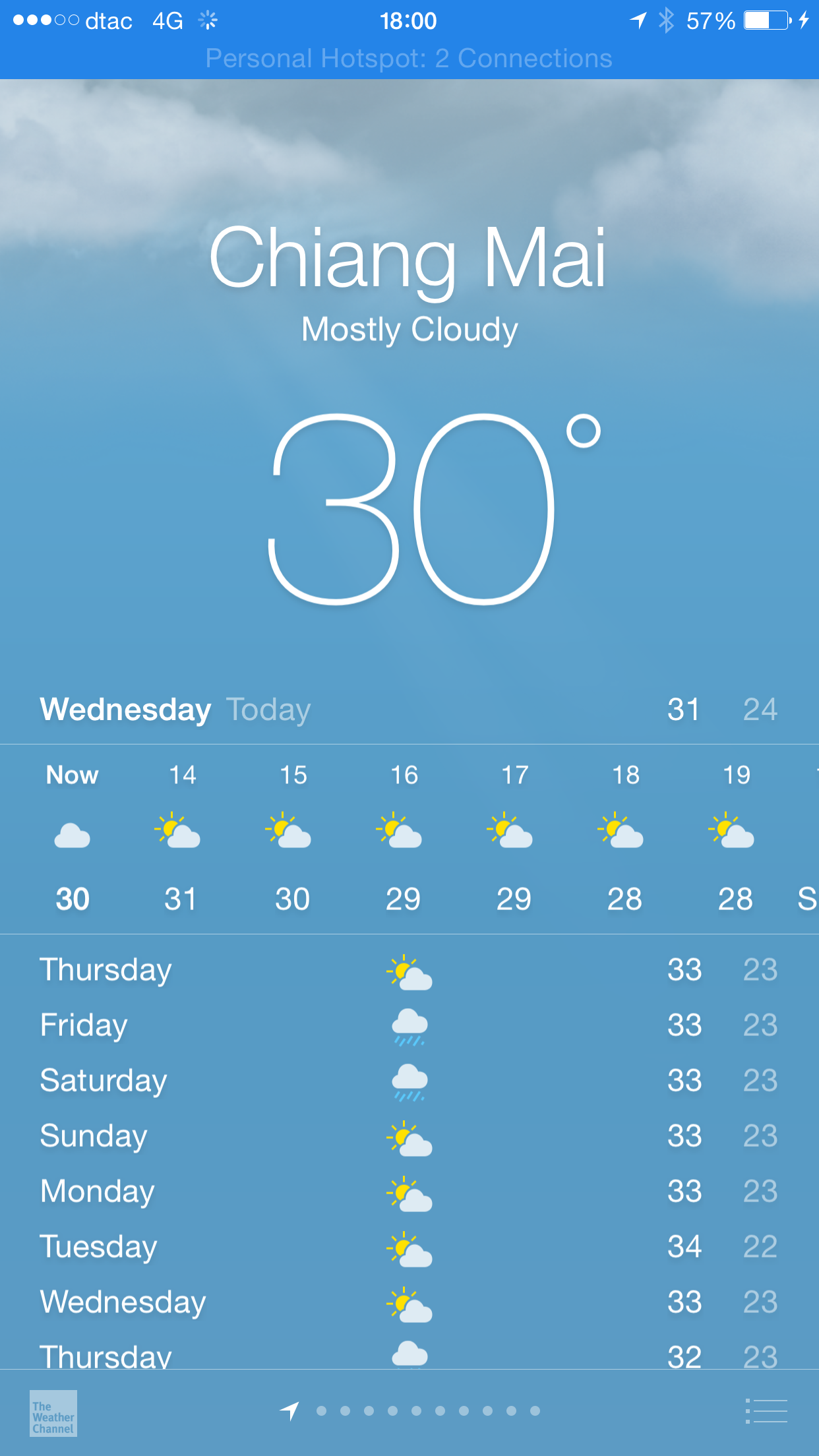This screenshot is taken from a smartphone, featuring a blue background with scattered clouds near the top. A blue border at the top displays the connectivity status as 4G and signal strength with five bubbles, three of which are filled in white, signifying good reception. The battery icon on the right side shows 57% charge remaining, colored in white.

On the home screen, the user is viewing a weather app for the city of Chiang Mai. The current weather is listed as mostly cloudy with a temperature of 30 degrees Celsius. The top section of the app also indicates that today is Wednesday. The forecast predicts a high of 31 degrees and a low of 24 degrees, suggesting that the rest of the day will be partly sunny.

Beneath today's weather information, the app displays the forecast for the upcoming week, spanning from Thursday to the following Thursday. Each day’s forecast is accompanied by an emoji representing the expected weather condition; for instance, Thursday is illustrated with a sun partially obscured by a cloud. High temperatures are shown in white, while low temperatures are depicted in a more grayish color.